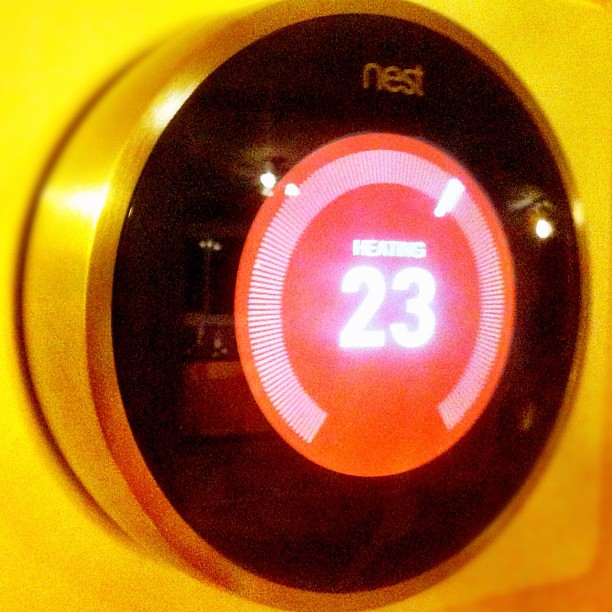The image showcases a Google Nest thermostat elegantly displayed against a warm, golden-yellow background. The thermostat features a circular, cylindrical design with a metallic, bronze-hued outer rim that visually recedes about half an inch to a matte black interface. Emblazoned in white at the top of the black circle is the brand name "Nest."

Prominently displayed on the central screen is a glowing numeral "23," indicating the current heating temperature setting. Surrounding this temperature readout, a sleek gauge allows users to adjust the climate control, with the knob positioned towards the upper right side of the display.

The sophisticated interface employs a gray electronic screen that enhances the visibility of the displayed information, making the numbers and icons stand out clearly. The photograph also captures subtle flash reflections on the black matte surface, suggesting that the photo was taken using a camera with a flash.

Overall, the Google Nest thermostat's high-tech and stylish design is highlighted by the image, portraying both its functional and aesthetic appeal.